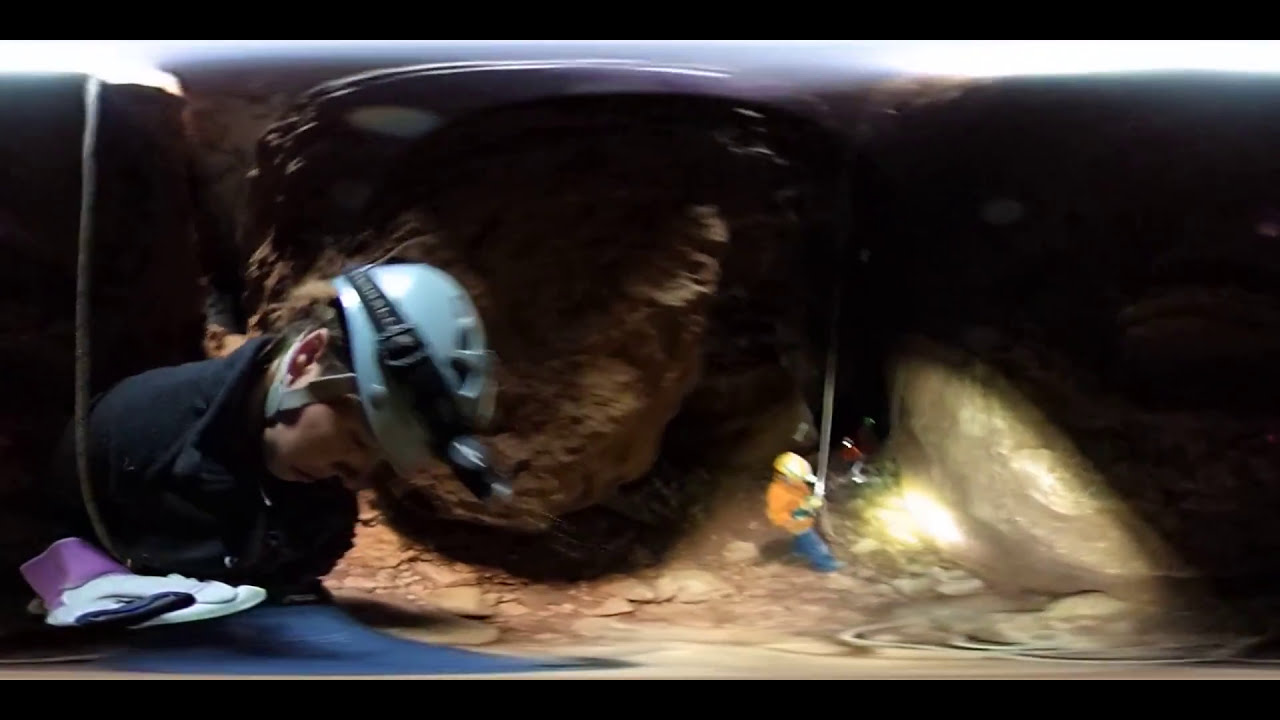The photograph, taken inside a dimly-lit cave, depicts a scene of two men seemingly involved in some form of excavation or mining work. In the foreground on the left, a man is visible from the bust up, wearing a black shirt and a light blue helmet with a non-illuminated flashlight attached. He is looking downward and appears to have white gloves on. His focused expression suggests concentration on a task. In the background, another man can be seen descending into the cave on a thick rope, indicating he is suspended from the cave's ceiling. This individual is dressed in an orange jacket, blue jeans, and a beige or yellow helmet with a very bright light that points directly at the large rock he examines. The surrounding environment features dusty, tan-brown rock formations typical of an underground cave, with partial illumination provided by the headlamp of the man in the background. The scene portrays a meticulous exploration or work activity within the rugged confines of the cave.